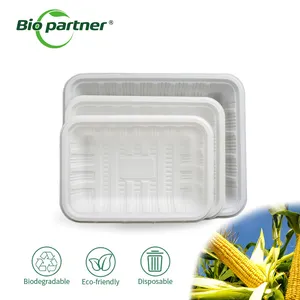The advertisement depicts eco-friendly, biodegradable, and disposable trays in focus. The image features a clean white background. In the upper left corner, a green logo reads “BioPartner,” indicating the company name. Central to the image are three trays of varying sizes—small, medium, and large—each with a textured, ribbed pattern to enhance grip and ease of cleaning. The trays are in hues of white or light gray. In the lower left, text emphasizes the trays' eco-friendly nature, with icons representing recyclability, a leaf for eco-friendliness, and a trash can for disposability. The lower right corner showcases an ear of corn growing under a brilliant blue sky, reinforcing the sustainability theme.